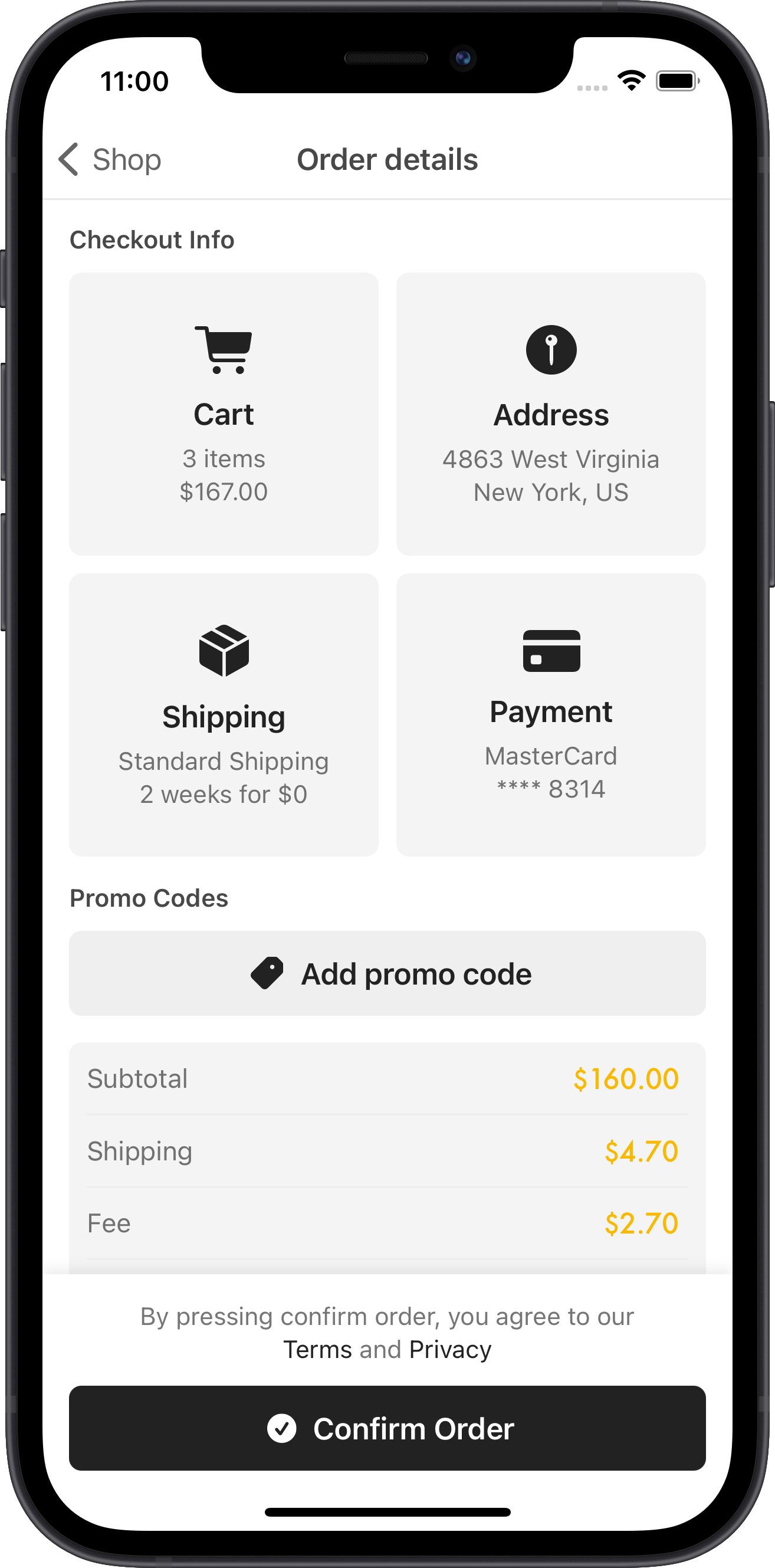The image depicts the checkout screen of a shopping app on an iPhone. At the top, there is a navigational arrow pointing to the left, labeled "Shop." Below it is the "Order Details" section, followed by "Checkout Info."

The first part of the Checkout Info displays a shopping cart icon with a label indicating "Cart (3 items) $167." Further down, the shipping address is listed as "48363 West Virginia, New York, U.S."

A shipping option is shown next, labeled as "Standard Shipping," with an estimated delivery time of two weeks and no additional cost for shipping. The payment section notes the last four digits of the user's credit card number.

There is also a section for entering promotional codes. Below that, the subtotal for the order is detailed as $160, with an additional shipping fee of $4.70 and a service fee of $20.76.

A note at the bottom specifies that by pressing "Confirm Order," the user agrees to the app's terms and privacy policy.

Finally, the "Confirm Order" button is prominently displayed in black with white letters and a checkmark next to it. The subtotal and related fees are highlighted in yellow, while the rest of the text is in black and gray. This screen serves as the final step for placing an order on the app.